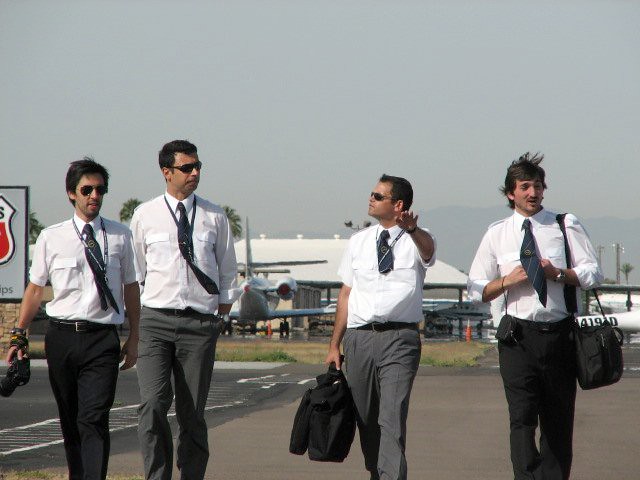The image depicts four men walking on a runway, surrounded by airplanes and a grassy background. They all appear to be wearing a uniform of white long-sleeve button-down shirts with blue or black ties and formal attire, including either gray or black dress pants. Two of the men have their shirt sleeves rolled up. The man in the middle is walking with one hand raised and holding a bag with the other, while the leftmost man carries a camera and the rightmost man also carries a bag. Three of the four men are wearing glasses. The weather is sunny, providing natural light to the scene, but the sky appears grayish and somewhat foggy, adding a distinct atmosphere to the image. The overall setting, with the large airplane in the background, suggests they might be pilots either preparing to board or having just disembarked from a plane.